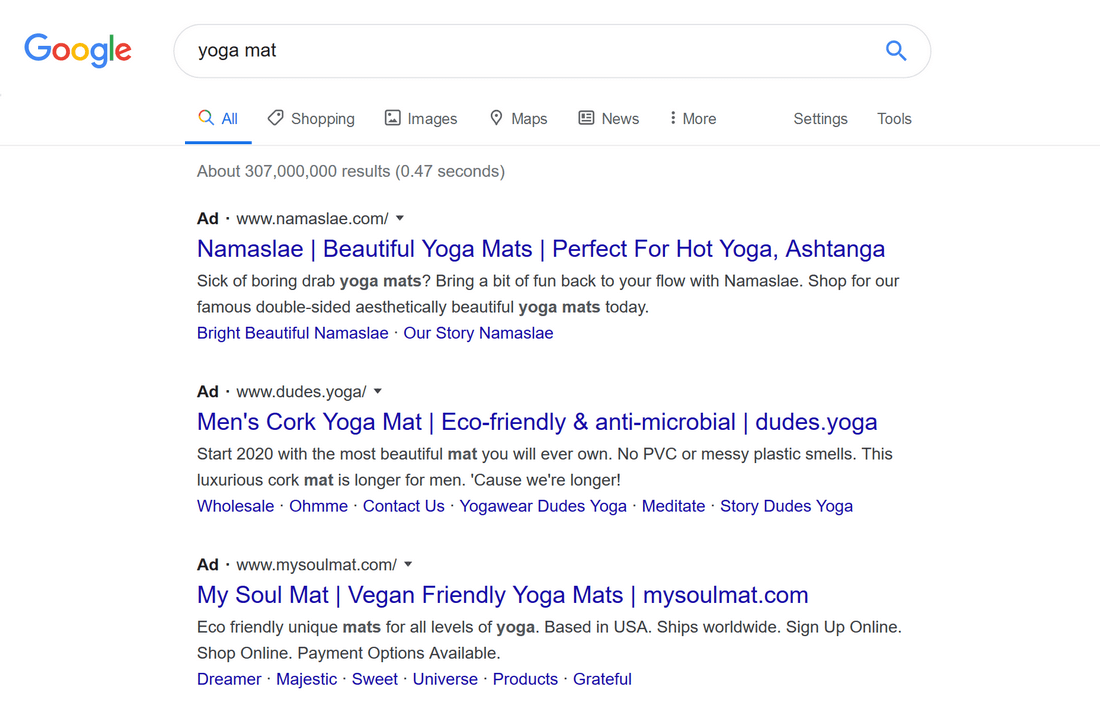**Image Description: Google Search Results for "Yoga Mat"**

The image depicts a Google search results page with the query "yoga mat" entered in the search bar. The background of the page is white, and the logo "Google" appears in the top left corner in its iconic colorful lettering. To the right of this logo, there is a white search bar outlined with a light gray border. The search terms "yoga mat" are displayed inside the bar in black text. Adjacent to the search bar, on the far right, is a bright blue magnifying glass search icon.

Below the search bar, there is a horizontal menu featuring search filter options in dark gray text. The options include "All," "Shopping," "Images," "Maps," "News," and "More"; additional options "Settings" and "Tools" appear on the far right. The word "All" is highlighted in bright blue and underlined, indicating the active filter. Just beneath this menu, a line of gray text indicates approximately 307 million results were found in 0.47 seconds.

The first search result is for Namaste Yoga Mats. The title, "Namaste - Beautiful Yoga Mats Perfect for Hot Yoga, Ashtanga," is displayed in bright blue text. The description beneath it, rendered in dark gray text, reads, "Sick of boring drab yoga mats? Bring a bit of fun back to your flow with Namaste. Shop for our famous double-sided aesthetically beautiful yoga mats today." Following this, in bright blue text, are links to additional pages: "Bright Beautiful Namaste," "Our Story," and "Namaste."

The second search result is for a men's cork yoga mat from the website dudes.yoga. The title, "Men's Cork Yoga Mat - Eco-Friendly and Antimicrobial," appears in bright blue text. The accompanying description, in gray text, states, "Start 2020 with the most beautiful mat you will ever own. No PVC or messy plastic smells. This luxurious cork mat is longer for men because we're longer!" Further available links in bright blue text are "Wholesale," "OHHMME," "Contact Us," "Yoga Wear," "Dudes.yoga," "Meditate," "Story," and "Dudes.yoga."

Below these entries, the search results continue with additional listings.